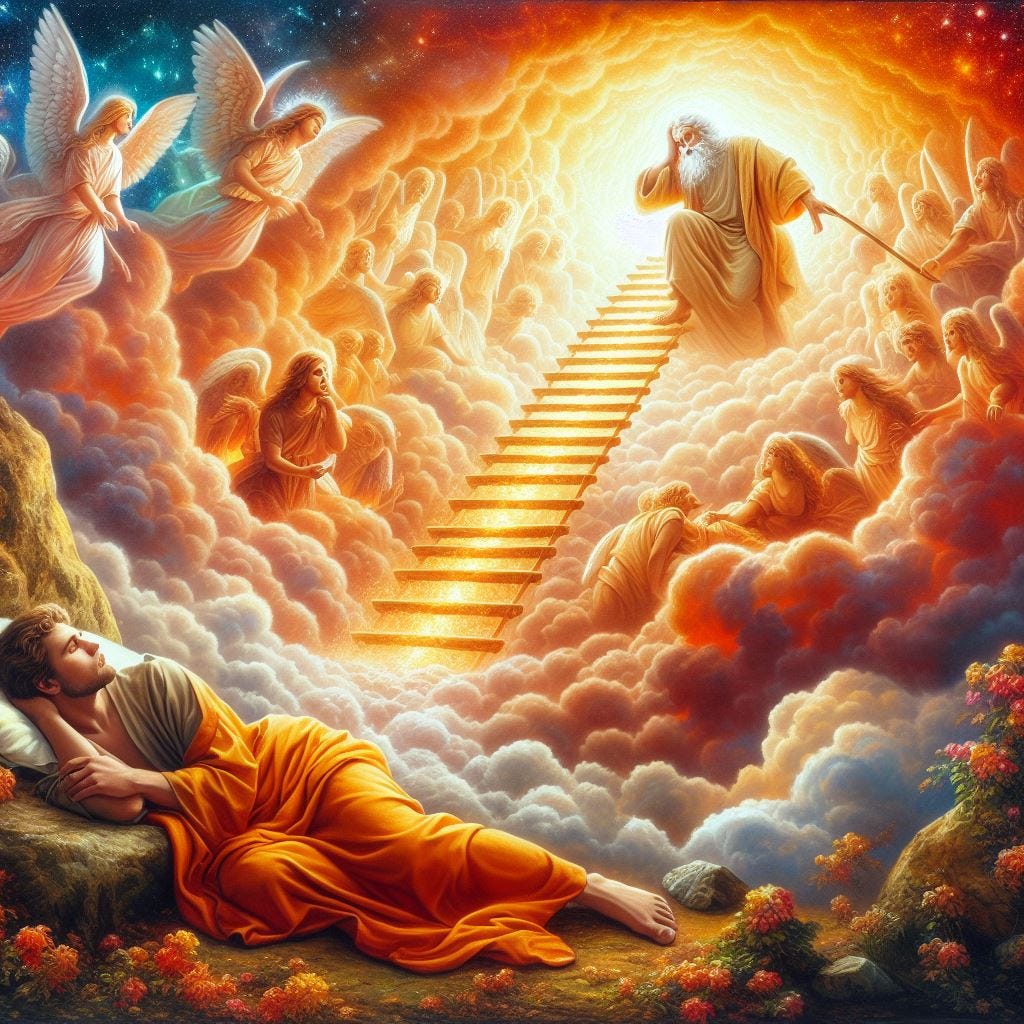In this religious artwork, we observe a vivid and captivating scene characterized by a blend of dark and bright hues. At the center, a golden ladder extends from a tunnel of clouds, bathed in radiant orange light that fades to a lighter hue towards the inside, suggesting a heavenly portal. Perched near the top of the ladder, an elderly man with a long white beard, dressed in a white robe and yellow cloak, holds a cane and rests one hand on his head. He is stepping out from the glowing tunnel, which is illuminated further by multiple angels.

The bottom landscape presents a rich outdoor setting with a young man lying on his side atop a rocky outcrop. He has light brown skin and hair, a slight beard, and is dressed in a light brown tunic partially covered by an orange blanket. His head rests on a pillow, and he gazes contemplatively towards the man on the ladder. The ground around him is dotted with marigold-like flowers, along with various yellow, pink, and red blooms.

The skies on the upper left show a darker, teal backdrop studded with stars, against which two angels with white bodies, long white wings, and yellow hair are flying. The entire image is a striking mixture of celestial and earthly elements, creating a mesmerizing vision of an ascent to the divine.